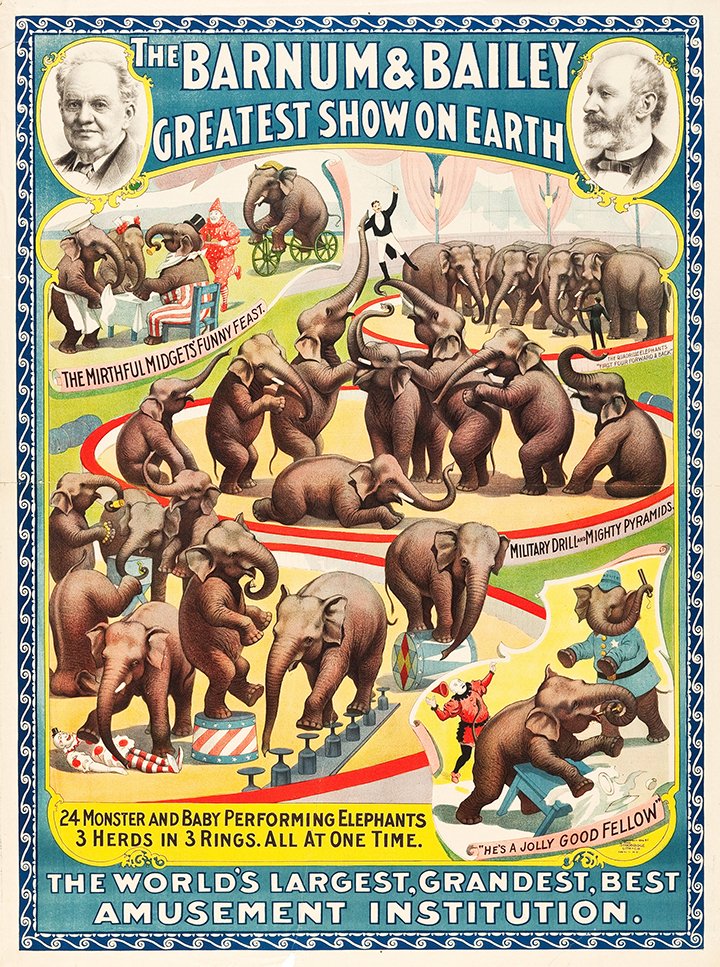This vibrant and detailed promotional poster for the Barnum and Bailey Circus, titled "The Greatest Show on Earth," captures the grandeur of this historic spectacle. The poster features images of the two founders: an older man with a disheveled horseshoe haircut occupies the upper left-hand corner, while the upper right-hand corner showcases a bald man with a salt-and-pepper beard. The header of the poster boasts "Barnum and Bailey Greatest Show on Earth" in bold white lettering against a light blue background, framed by a white wave-patterned banner.

Elephants dominate the central imagery, showcased in a variety of extraordinary acts. Some elephants are impressively riding bicycles while others stand upright, lifting circus performers with their trunks. A whimsical scene features a clown approaching a table where elephants are gathered. Notable banners throughout the poster highlight key attractions, such as "The Mirthful Midgets Funny Feast," "Military Drill and Mighty Pyramids," and "He's a Jolly Good Fellow." The poster further promises "24 Monster and Baby Performing Elephants, Three Herds and Three Rings All at One Time."

The footer proudly declares it as "The World's Largest, Grandest, Best Amusement Institution," enveloping the claims and inviting viewers into an unparalleled world of entertainment. The rich array of images and proclamations illustrate the dynamic circus acts, positioning Barnum and Bailey as the epitome of amusement and wonder.